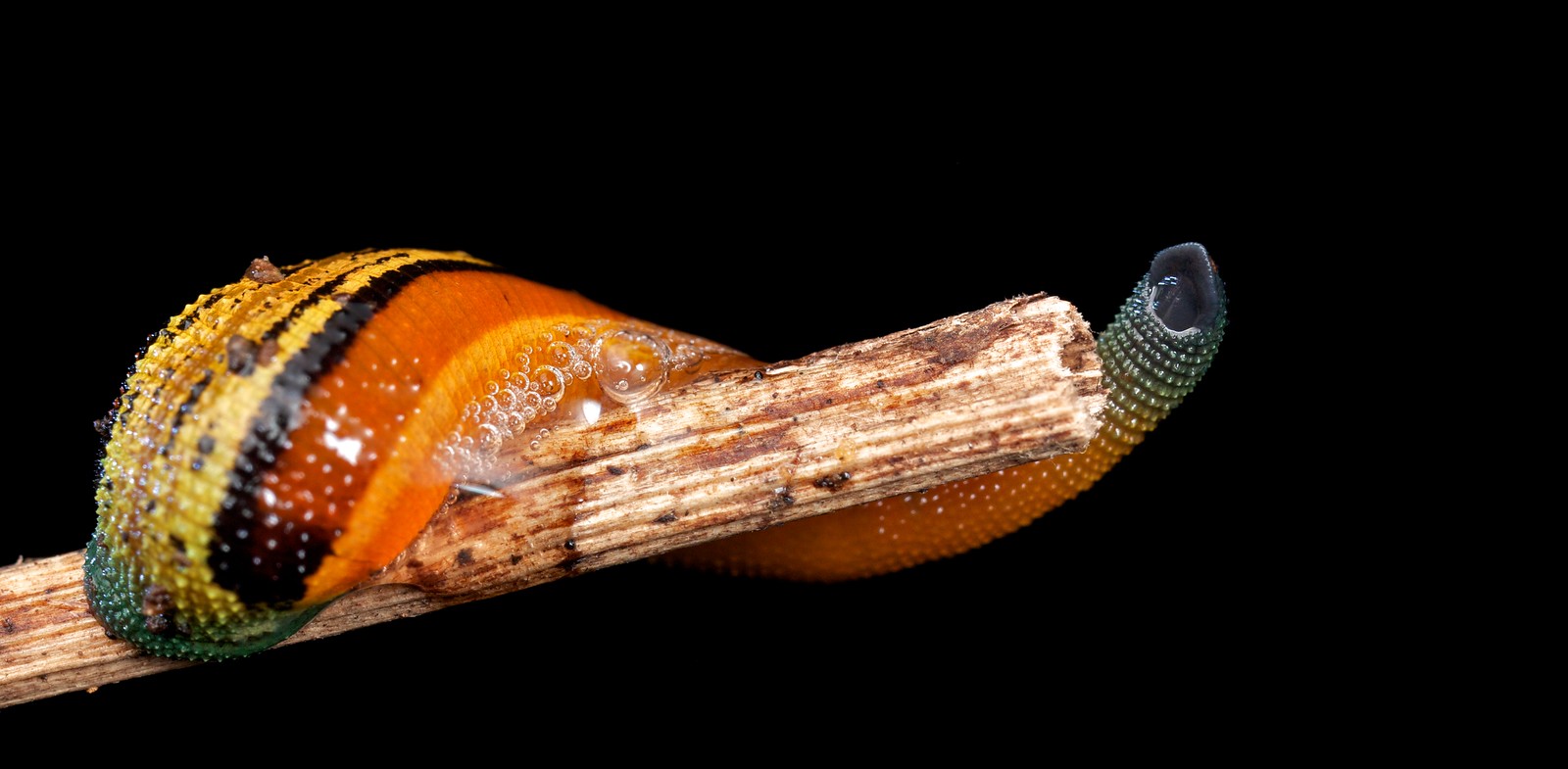In a photograph set against an utterly black background, a richly colored slug intricately wraps around a woody, bamboo-like branch that extends from the bottom left towards the center of the image. The slug's body showcases a vibrant array of colors, with striking green, yellow, orange, and black stripes running along its length. The critter's slimy exterior, accentuated by sparkling water bubbles scattered on and around it, hints at an underwater setting. The slug's right side glows with a mix of orange and yellow hues, while darker black and green tones mark the left end. A notable large opening, possibly an eye, is wrapped in a grayish hood, adding an intriguing focal point. The detailed texture and sliminess of the slug, juxtaposed with the rugged, broken piece of wood, create a stark and captivating contrast against the dark void of the background.